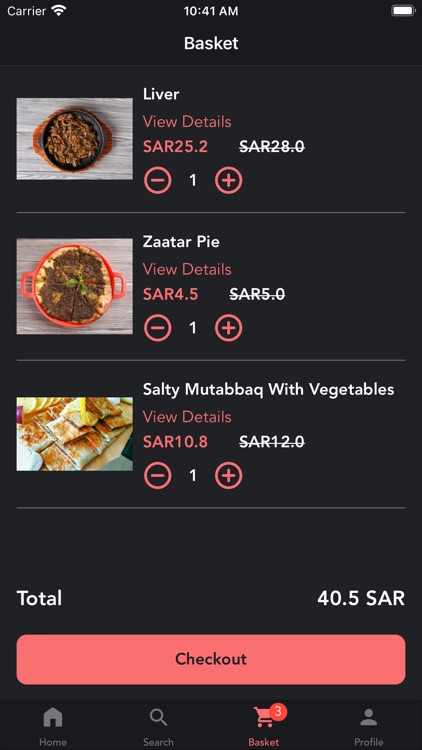This image depicts a smartphone screen displaying a food ordering app's webpage. The current time is 10:41 AM, and the phone's battery is almost fully charged while connected to a WiFi network. The user is viewing the "Basket" section of the app, which contains three food items. The first item is liver priced at SAR 25.2, the second is a za'atar pie costing SAR 4.5, and the third is a salty mutabak with vegetables priced at SAR 10.8. Each item is listed with a quantity of one in the basket, bringing the total amount to SAR 40.5. The screen also features a prominent red "Check Out" button for proceeding with the purchase. At the bottom of the app interface, there are navigation options: "Home," "Search," "Basket" (currently active), and "Profile."